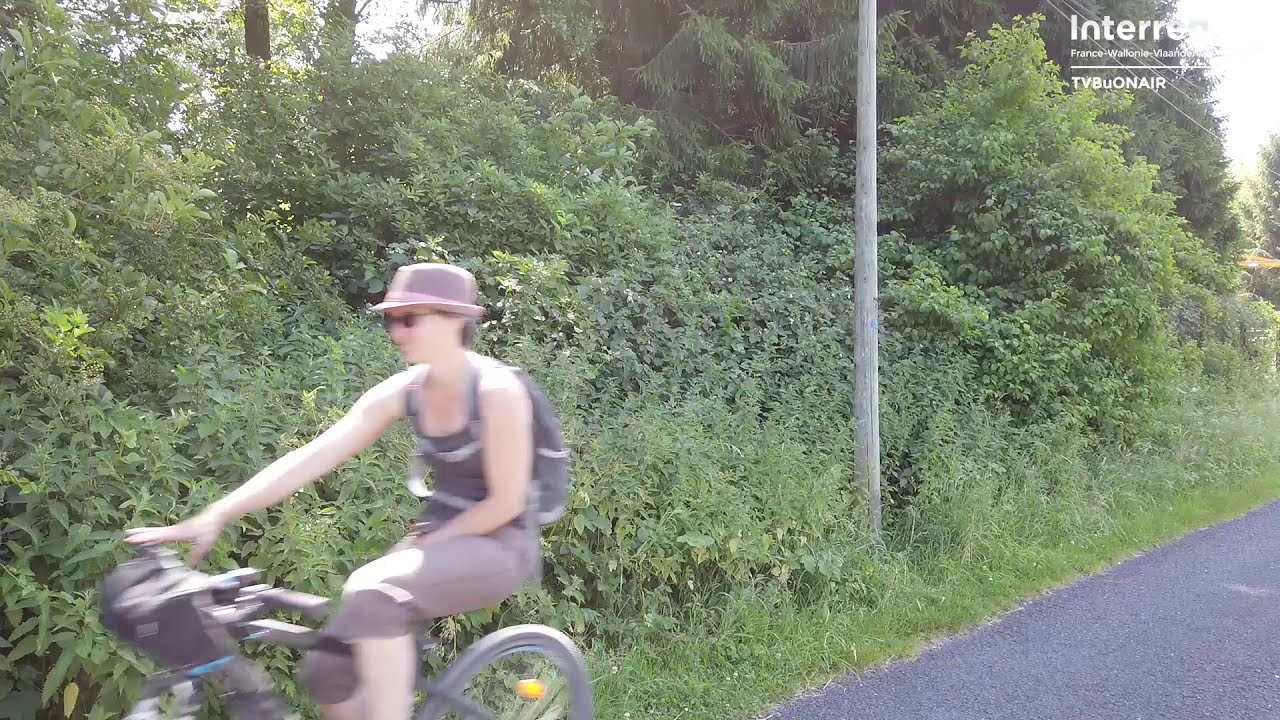The bright daytime photograph captures a person, likely female, riding a gray bicycle. The cyclist, adorned with a hat, sunglasses, and gray attire consisting of a tank top and shorts, appears blurred due to motion, suggesting a brisk pace. She's in the left portion of the image, while the bicycle's wheels almost touch the lower left corner. The paved, slate-colored road is evident at the bottom right corner, leading towards a dense woodsy area featuring lush green bushes and several trees. A telephone pole can also be observed behind her. In the top right corner, white text reads "INTERRERE" with additional lines showing "France-Wallany" and "TVBU on air," suggesting some sort of French broadcast.